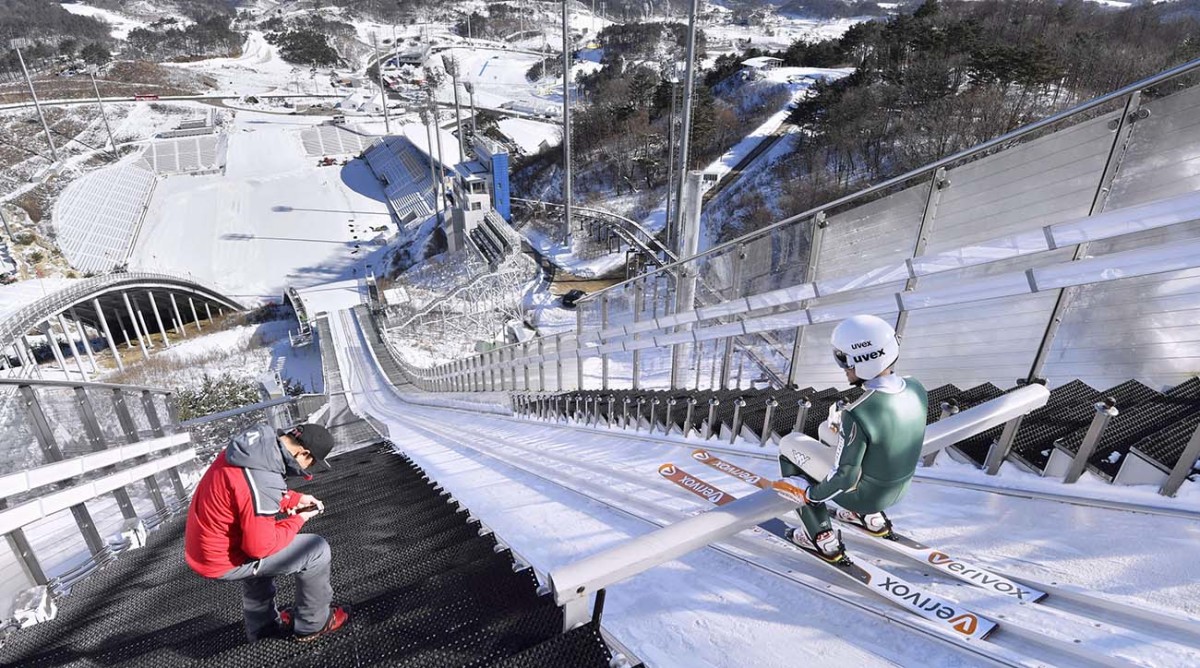In this detailed color photograph taken in landscape orientation, the viewer is positioned just behind and slightly to the left of a ski jumper perched at the top of an extremely steep and high ski jump ramp. The skier sits on a crossbar, holding himself steady to prevent an early descent. He is clad in a tight, green and white ski outfit and a white helmet, with his skis nestled in tracks that guide the jump. To the left of the skier, positioned on black stairs that run along the ramp's edge, stands an official dressed in a red jacket with a gray hood, gray pants, and a black cap. The official is kneeling down, diligently noting something on a clipboard. The photograph captures the stark contrast of the white ramp against the black steps, extending down to a small, snow-covered landing area, with a snowy landscape stretching into the background. The composition evokes a sense of the vast height and tension of the impending jump.